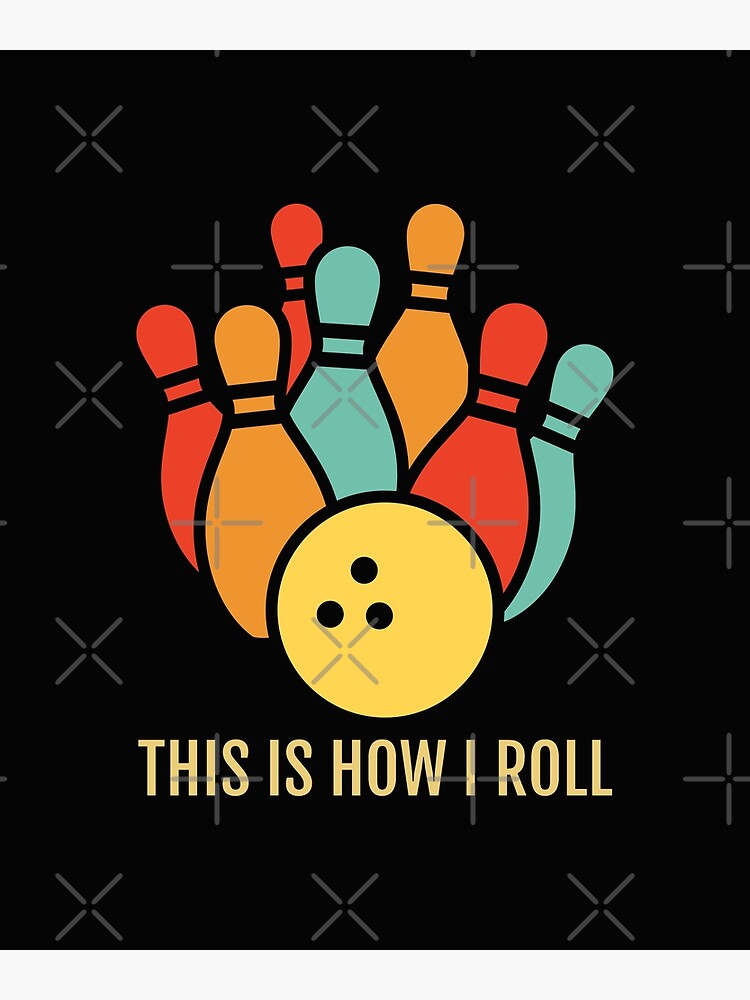This image features a vivid, cartoonish depiction of a bowling scene with a black poster-esque background. At its center are seven bowling pins, arranged in a tight cluster and painted in a variety of vibrant colors: three red, two light blue, and two light orange. These pins have distinctive black stripes around their necks. In front of them is a bright yellow bowling ball with the characteristic three finger holes. Beneath the image, bold yellow capital letters declare, "THIS IS HOW I ROLL." The backdrop is decorated with evenly spaced gray X's and crosses, forming a grid-like pattern across the black surface. The overall design suggests it could be suitable for a t-shirt, flyer, or other promotional material, capturing the playful spirit of bowling.